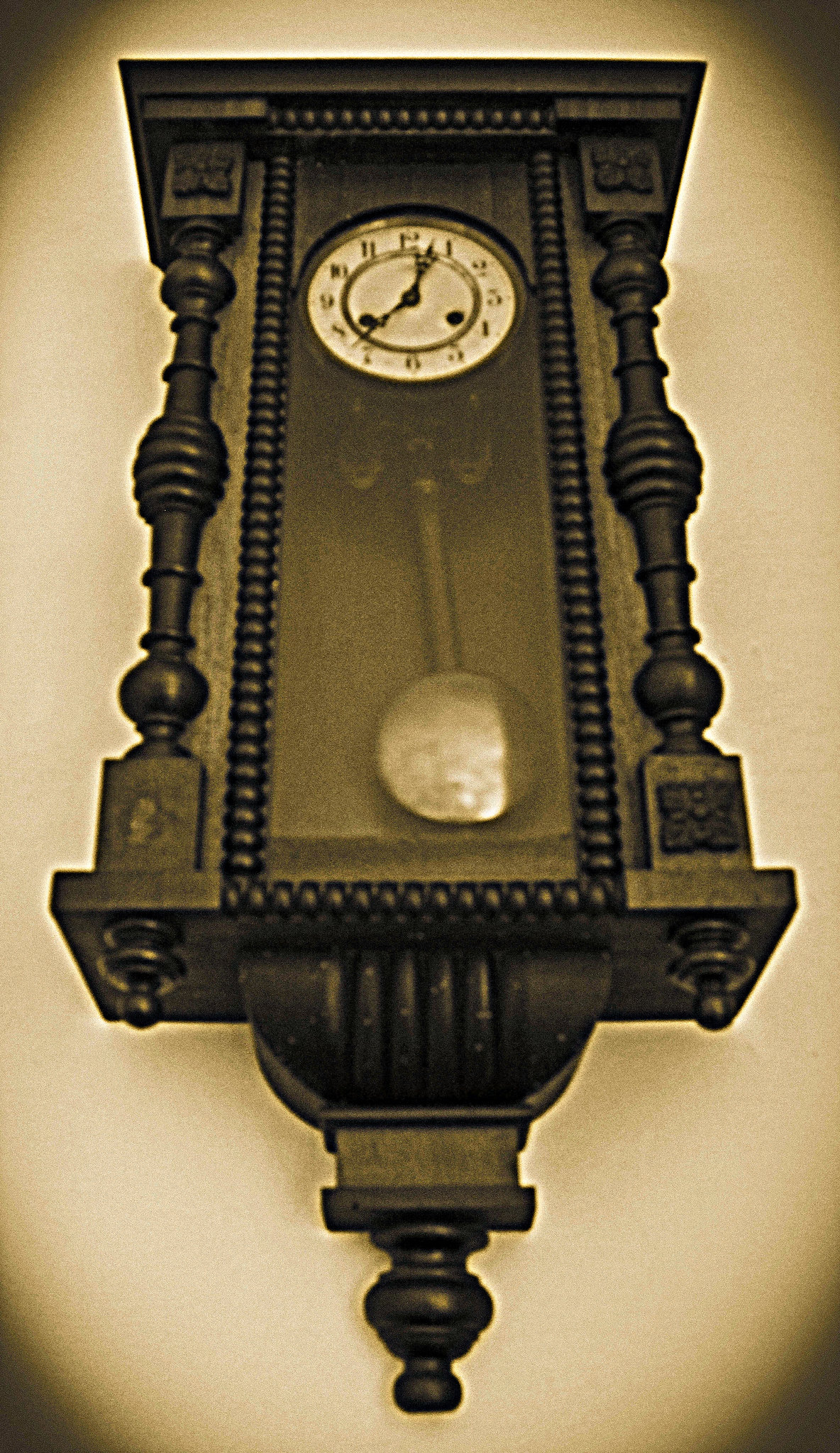The photograph is a color image with an aged, sepia-toned effect, giving it a nostalgic black-and-white appearance with a yellowish hue. The subject is an old-fashioned wooden clock, viewed from a low angle on a wall, surrounded by darkened, shadowy edges. The clock features a round, silver face with black numerals and two black hands indicating the time as approximately 12:40. Below the clock face is a silver pendulum, positioned to the right. The clock itself is encased in a long, rectangular glass enclosure adorned with a series of small circular details along the dark border. Flanking the sides of the clock are ornate decorative pillars. Additionally, there are two balcony-like structures—one situated above and one below the main clock body. The clock's base tapers into a curved, multi-layered section that is significantly narrower than the central part of the clock, enhancing the antique elegance of the piece.